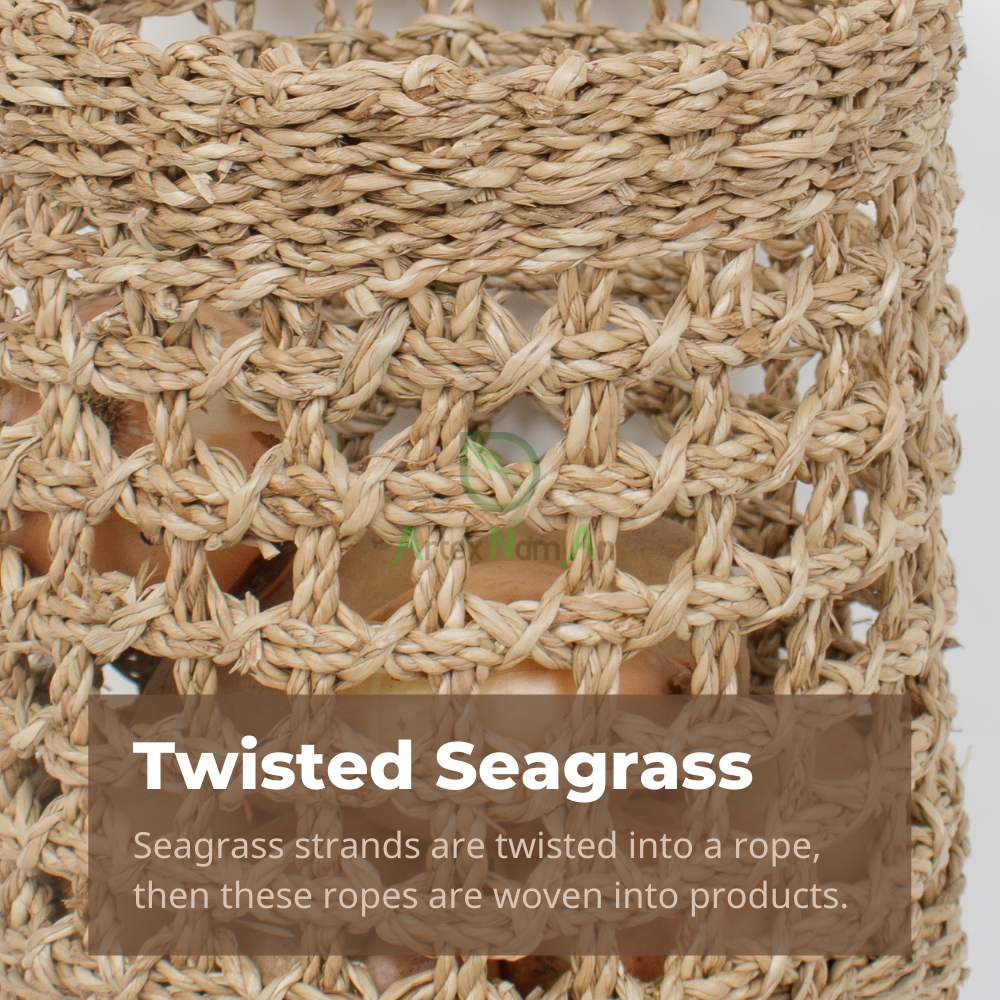The image depicts a close-up view of a basket or hamper made from twisted seagrass ropes intricately woven together to create a lattice-like structure. The seagrass strands are knotted and interwoven, forming a thick band at the top, with visible gaps between the strands. Inside the basket, there appear to be items, possibly onions or small packages, though the exact contents are not clearly discernible. At the bottom of the image, there is a brown rectangular text box with white lettering that reads "Twisted Seagrass," and below it in a lighter brown font, it explains, "Seagrass strands are twisted into ropes and these ropes are woven into products." In the center of the image, a green and gray watermark is visible, bearing the text "ARTEX NAMAN," with the letters A, N, and A highlighted in green. The background of the image is plain white, emphasizing the detailed texture and craftsmanship of the woven seagrass basket.